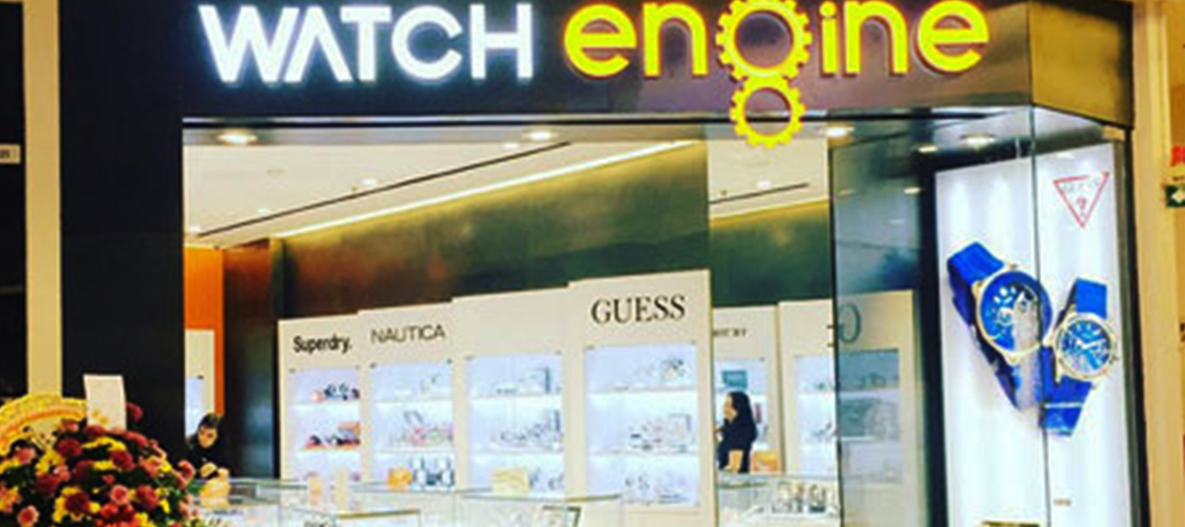In this image, we are peering through the window of a watch shop set within a bustling mall. The entrance to the store is framed by a prominent banner that reads "Watch Engine," creating an inviting threshold. Just outside the entrance on the left, there is a vibrant bouquet of purple, yellow, and green flowers, accompanied by a small post-it sign. Stepping into the store, the interior is dotted with several panels showcasing different watch brands, including Nautica and Guess, while another brand name, Sierbinski, appears on one of the displays. 

On the right side of the window, a large advertisement exhibits a selection of men’s and women's watches, prominently featuring a blue and gold watch against a white background. The store’s aesthetic intertwines black and white elements, complemented by touches of tan, red, and other subtle hues from the various products and decorations. 

Inside the shop, a man is seen leaning on the counter situated at the lower left of the picture, creating a sense of activity and human presence. Various tables and product rows, although somewhat indistinct, are arranged around the space, suggesting a well-stocked retail environment. Overall, the scene captures the inviting and meticulously organized ambiance of a modern watch shop within a mall.